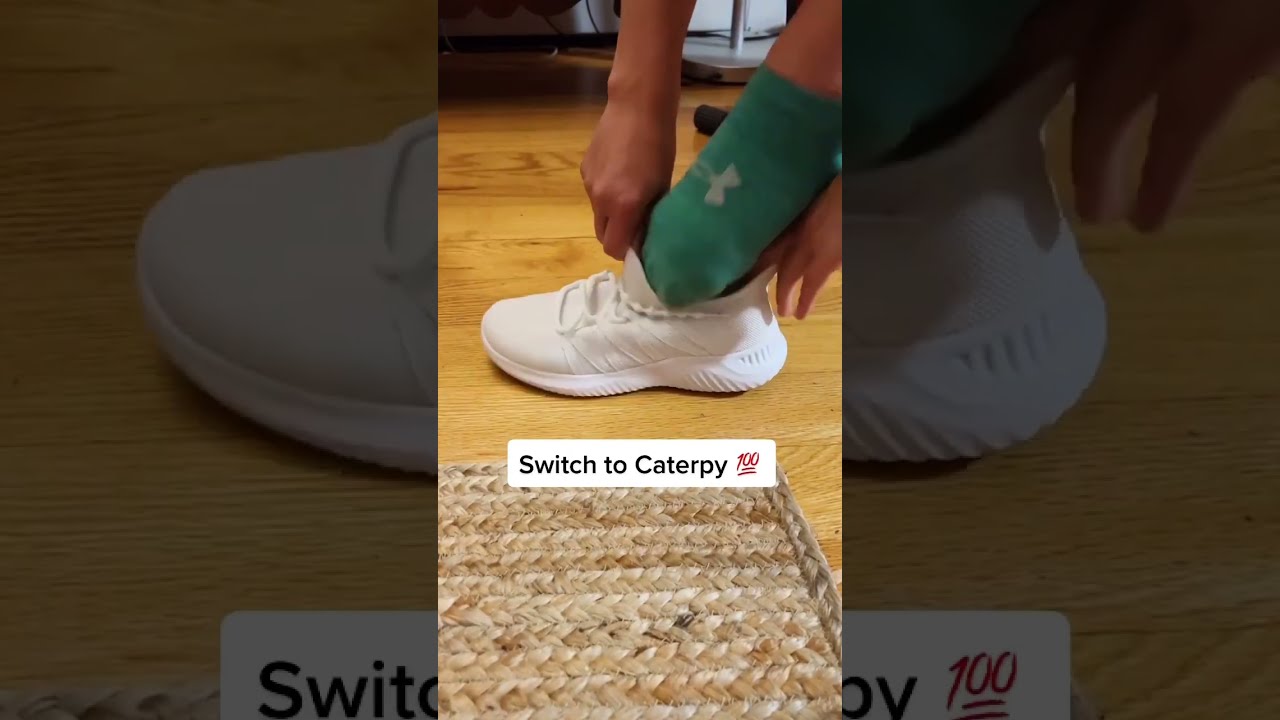This high-definition photograph captures a close-up scene of an individual putting on a white sneaker. The central focus is a yellow-green sock-adorned foot, with the sock featuring a gray Under Armour logo. The person's light brown hands can be seen working to fit the foot into the all-white athletic shoe. The action takes place on a beige wood floor, complemented by a brown rattan braided rug placed nearby.

The photographic composition includes an intriguing design where the central image is bordered on the left and right by enlarged, faded, close-up sections of the same sneaker. The indicated text, "Switch to Canterpie," in black and the red number "100" add a unique element to the middle of the image.

In essence, the visual not only captures the moment of putting on the sneaker but also artistically enhances the scene with a mirrored, shaded border that focuses on the shoe, bringing attention and depth to the central action.